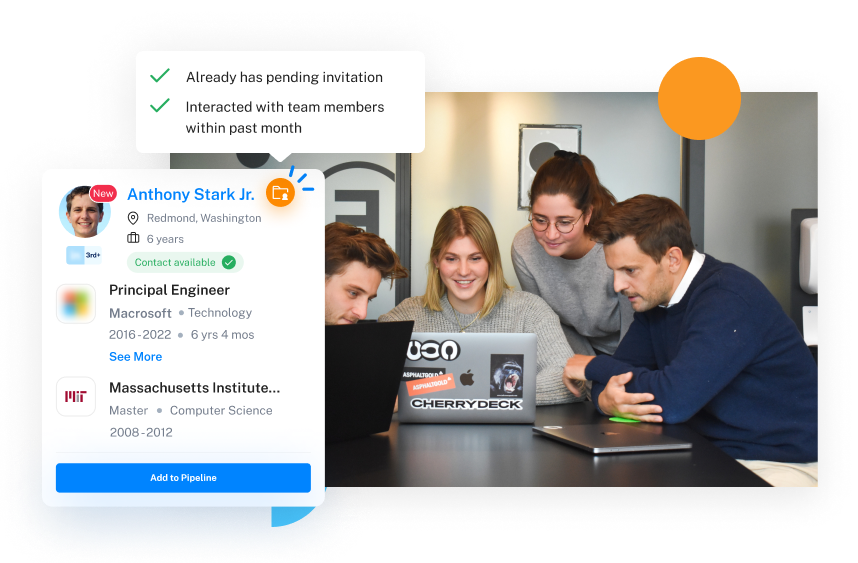In this image, you see four people gathered around a workspace, focused on their laptops. They appear to be collaborating or working on a project together. The group consists of two men and two women. One of the women, who is standing and wearing a pair of glasses, seems to be addressing the group. The other three individuals are seated, each with a laptop in front of them. The laptops are a mix of silver MacBooks and black laptops.

On the wall behind them, text detailing a professional profile is visible. It reads: "Anthony Stark Jr., Redmond, Washington. Six years of experience. Contact available. Principal engineer at Microsoft Technology from 2016 to 2022. Six years and four months tenure. Education includes a Master of Computer Science from the Massachusetts Institute of Technology, 2008 to 2012." 

The man seated to the right is dressed casually in a blue sweater over a white t-shirt. The setting likely represents a collaborative working environment, possibly a meeting or brainstorming session among tech professionals.